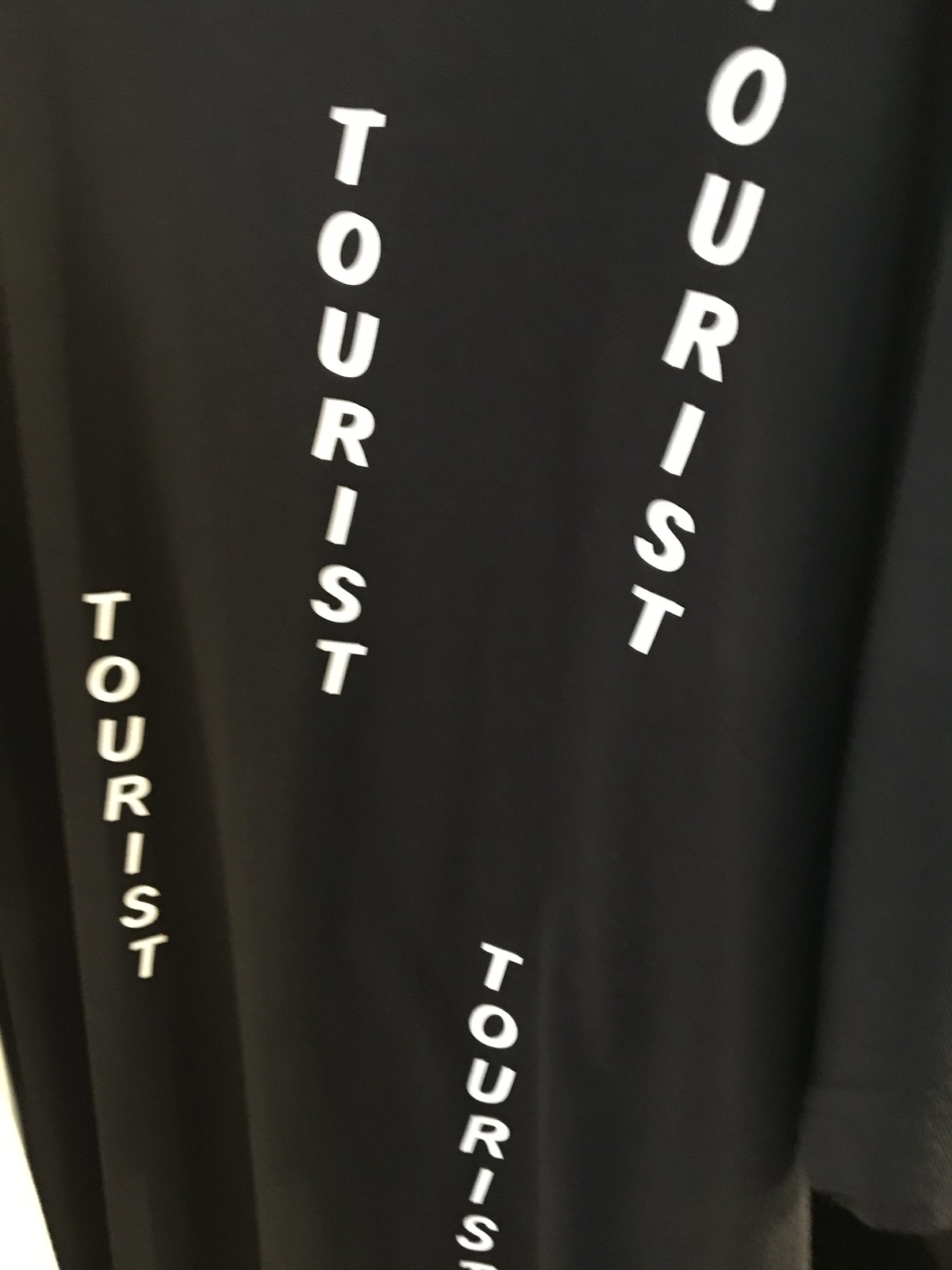This image features a close-up view of a black, long-sleeve shirt or robe, captured from the shoulders down to just below the neckline. The fabric showcases soft, natural folds, with varying light reflections accentuating the texture. Although the hem is not visible, the sleeve cuff can be seen, implying the garment's length up to a certain point. This shirt, which is draped on a hanger, prominently displays the word "TOURIST" printed vertically in four separate locations across the front in bold, white capital letters. The background is a solid, deeper black, creating a stark contrast that emphasizes the shirt's design. The lighting appears to originate from the right side, with subtle reflections highlighting the lower portion of the garment.